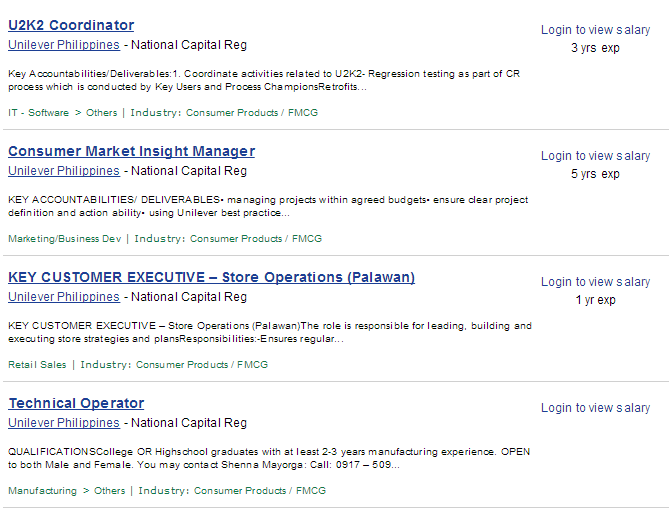**Job Openings in the National Capital Region**

This is a detailed list of job openings available at Unilever Philippines in the National Capital Region. Each position is presented with its job title in bold dark blue text. Below is a structured description:

1. **U2K2 Coordinator**
   - **Company:** Unilever Philippines
   - **Location:** National Capital Region
   - **Key Accountabilities/Deliverables:** 
     - Coordinate activities related to U2K2 regression testing as part of a CR process conducted by key users and process champions.
   - **Industry:** IT-Software, Consumer Products/FMCG (in green text)
   - **Experience Required:** 3 years
   - **Additional Info:** Login to view salary

2. **Consumer Market Insight Manager**
   - **Company:** Unilever Philippines
   - **Location:** National Capital Region
   - **Key Accountabilities/Deliverables:** 
     - Manage projects within agreed budgets.
     - Ensure clear project definition and actionability using Unilever best practices.
   - **Department:** Marketing/Business Development
   - **Industry:** Consumer Products/FMCG
   - **Experience Required:** 5 years
   - **Additional Info:** Login to view salary

3. **Key Customer Executive - Store Operations (Palawan)**
   - **Company:** Unilever Philippines
   - **Location:** National Capital Region
   - **Responsibilities:** 
     - Lead, build, and execute store strategies and plans.
     - Ensure regular operations and advancements in store strategies.
   - **Department:** Retail Sales
   - **Industry:** Consumer Products/FMCG
   - **Experience Required:** 1 year
   - **Additional Info:** Login to view salary

4. **Technical Operator**
   - **Company:** Unilever Philippines
   - **Location:** National Capital Region
   - **Qualifications:** 
     - College or high school graduate with at least 2-3 years of manufacturing experience.
     - Open to both male and female candidates.
     - Contact: Shanna Mayorga (Call 0917-509....)
   - **Department:** Manufacturing
   - **Industry:** Consumer Products/FMCG
   - **Additional Info:** Login to view salary

Each job listing is accompanied by a horizontal gray line to help delineate between different postings. Detailed role responsibilities and required qualifications are provided to ensure candidates understand the expectations and criteria for each position.